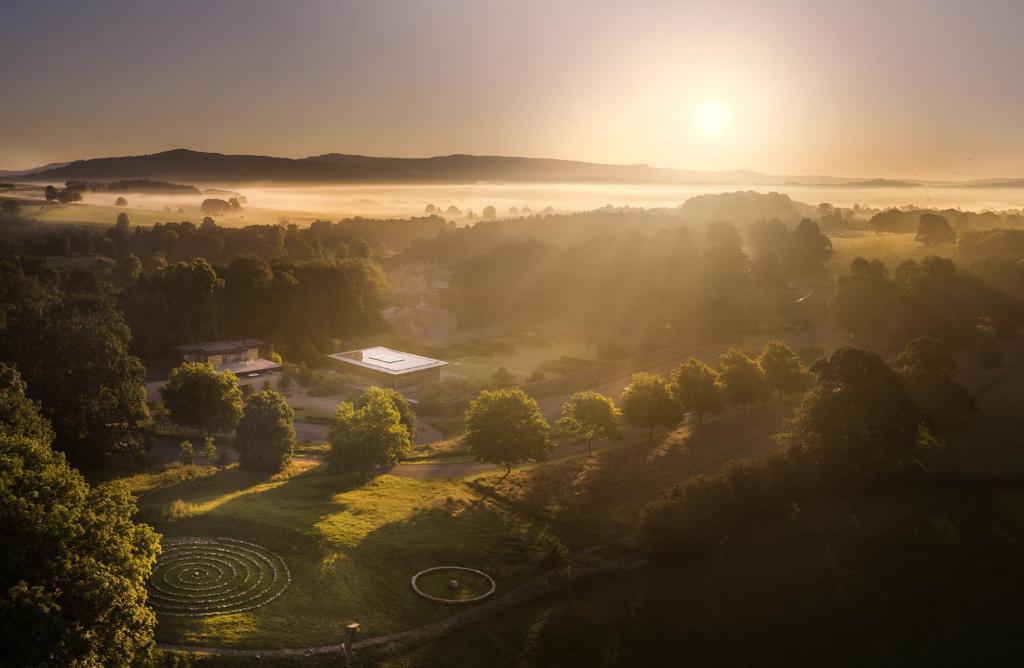An aerial photograph captures a serene landscape bathed in the golden hues of sunset. In the central left portion of the image, a modest house stands alongside a secondary building, possibly a garage, accessible via a winding road. The foreground features lush green fields interspersed with trees, some arranged in neat rows. A prominent white spiral, likely made of stones, stands out in the lower left corner of the grassy expanse. A smaller circle of stones with a sphere at its center is situated to the right of the spiral. The horizon reveals sloping mountains cloaked in a soft, foggy mist, adding depth to the scene. The setting sun, low above the horizon, tinges the sky with a light, hazy yellow, casting a warm glow across the tranquil surroundings.